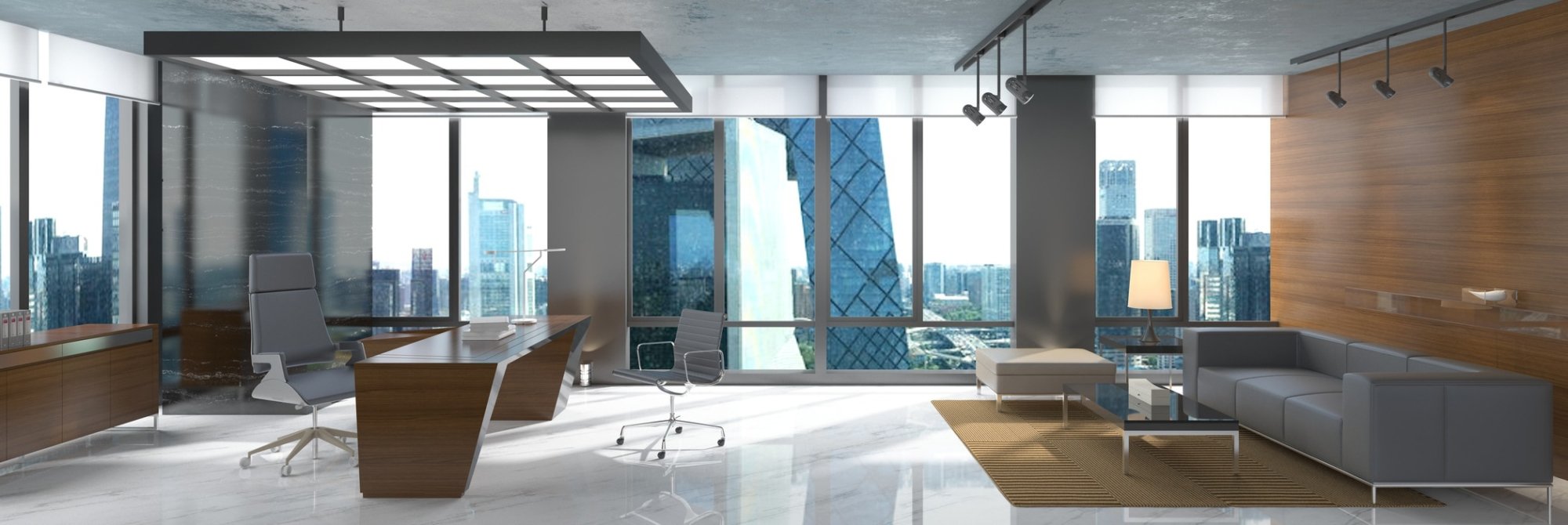Spacious and elegant, this large office room is adorned with modern Swedish-style furnishings. A central brown desk takes the spotlight, accompanied by a complementary lower bureau of the same hue. The seating includes a sophisticated grey leather chair and a matching grey couch, perfectly positioned on a plush brown rug. Massive picture windows dominate one wall, framed by sleek grey poles arranged both vertically and horizontally, offering breathtaking views of towering skyscrapers. Among the architectural marvels visible through the window is a mirrored sculpture or building, adding a touch of intrigue to the urban landscape. A small lamp and an ottoman beside the couch complete the room's stylish yet functional decor.